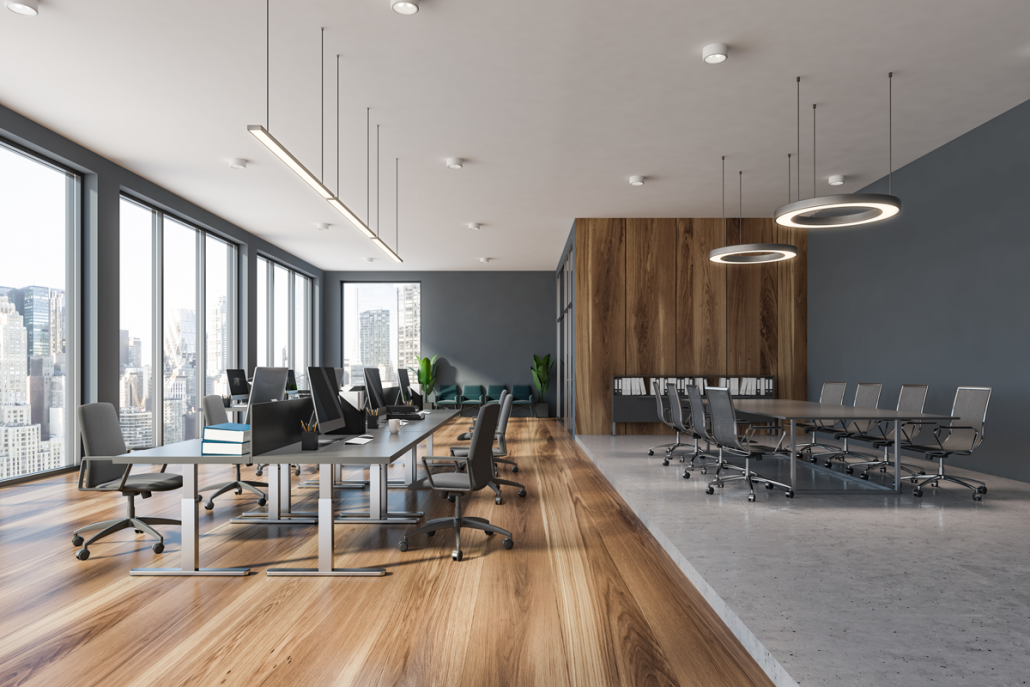The image depicts an upscale, modern office space with a sleek, minimalistic design. To the left, there are large floor-to-ceiling windows that offer a panoramic view of a cityscape, featuring skyscrapers, apartment buildings, and office complexes, indicating the office is situated on a high floor. Adjacent to these windows, the area is paved with polished hardwood floors and houses a large workstation. This workstation consists of long gray tables with multiple computer monitors, likely Macs, accompanied by office chairs on wheels. On the tables are various office supplies, including a couple of large blue books and jars filled with pens and pencils.

The right side of the image features a contrasting section with marble flooring, likely designated for meetings. Here, a substantial gray table is surrounded by eight metal office chairs, four on each side, beneath ring-shaped, disk-like office lights. This section exudes a high-end, professional ambiance suitable for boardroom discussions. In the background of this area, there is a blue seating area against the wall, possibly functioning as a waiting area, along with a bookshelf. The office has gray walls and a white ceiling, enhancing its bright and airy feel due to the abundant natural light streaming in through the generous windows, underscoring the space's modern and youthful aesthetic.